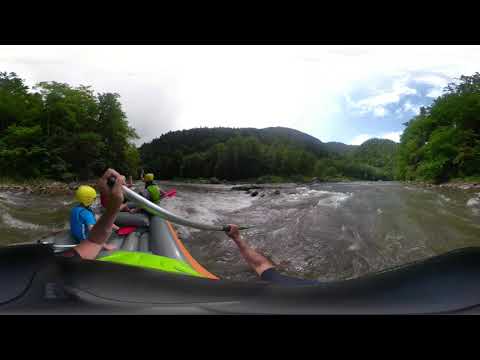This panorama photograph captures the exhilarating experience of river rafting from the perspective of a life raft navigating whitewater rapids. The image is cropped by thick black rectangles at the top and bottom. The upper half reveals a sky, predominantly white with patches of blue, especially cloudy to the right. The horizon line is dominated by tall, thick green pine trees, with a mountain range rising behind them. 

Below the horizon lies the foamy, bluish dark green river, churning with whitewater. On the image's left side, an orange and gray life raft can be seen, occupied by a group of four people wearing helmets and protective gear of various colors, like blue and green. One man, likely positioned at the back of the raft, grips a silver oar that's visibly bending under the force of the water. The action is intensified by the oar’s dynamic curve as it slices through the turbulent river, suggesting the photographer is also one of the rafters. The scene hints at a fork in the river, with the raft taking the more challenging left path, while a calmer stream flows to the right. The overall ambiance is one of adventure and thrill, with the bright, sunny weather highlighting the natural beauty and intensity of the rafting experience.